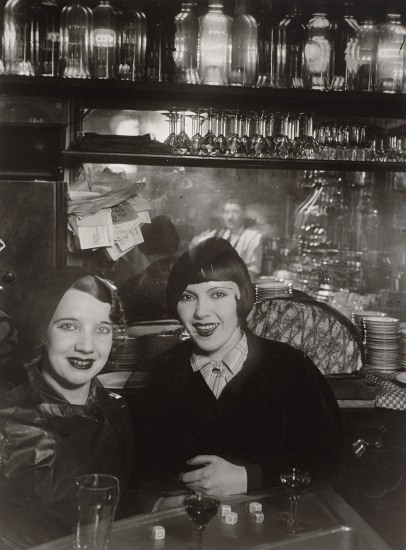This black and white photograph, likely from the 1920s or 30s, features two young women sitting at a bar counter. Both women are smiling at the camera, exuding a sense of camaraderie. The woman on the left is dressed in dark clothing, including a black hoodie-like jacket, and has lipstick on with dark hair visible under what might be a hood or bonnet. The woman on the right sports short dark hair, a black jacket, and a collared white shirt. They are seated at a table adorned with dice, a clear glass, and two martini glasses containing a dark drink.

In the background, there are multiple shelves stocked with various sizes of glass containers, including bottles and inverted wine glasses. There's also a mirror, which reflects a mustachioed bartender in a white shirt. The reflection also captures the back of the woman on the right’s head, suggesting that the man may be the photographer. Additionally, a suggestion box with papers sticking out can be seen on the left side in the mirror. The setting, detailed with miscellaneous items, plates, and other bar paraphernalia, creates an authentic glimpse into a bygone era.